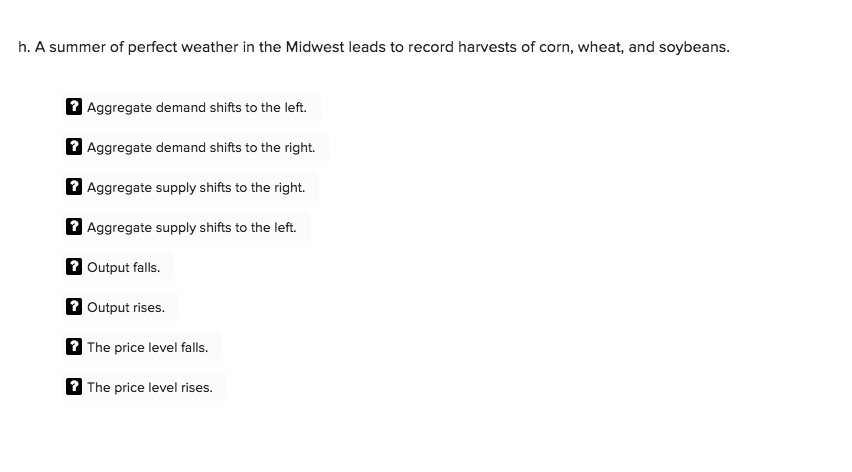The image is a monochromatic, black-and-white document containing a list of economic terms and annotations. It features a clean, white background without any border. At the top, aligned horizontally in the upper left corner, is a lowercase "h" followed by a period. Alongside this initial text, extending across the top, is the phrase: "A summer of perfect weather in the Midwest leads to record harvests of corn, wheat, and soybeans."

Immediately below this phrase, there are eight question marks, each set within individual black square backgrounds, creating a stark contrast with their white text. Adjacent to these question marks is a list of eight lines of text, all presented in a subtle, dark gray-to-black small font. These lines of text read, from top to bottom:
1. Aggregate demand shifts to the left
2. Aggregate demand shifts to the right
3. Aggregate supply shifts to the right
4. Aggregate supply shifts to the left
5. Output falls
6. Output rises
7. The price level falls
8. The price level rises

This vertically arranged list is indented slightly from the left margin, while the top line containing "h." is marginally shifted to the left compared to the subsequent column of text and question marks. The entire composition is rendered in shades of black, gray, and white, contributing to its stark and simple aesthetic.